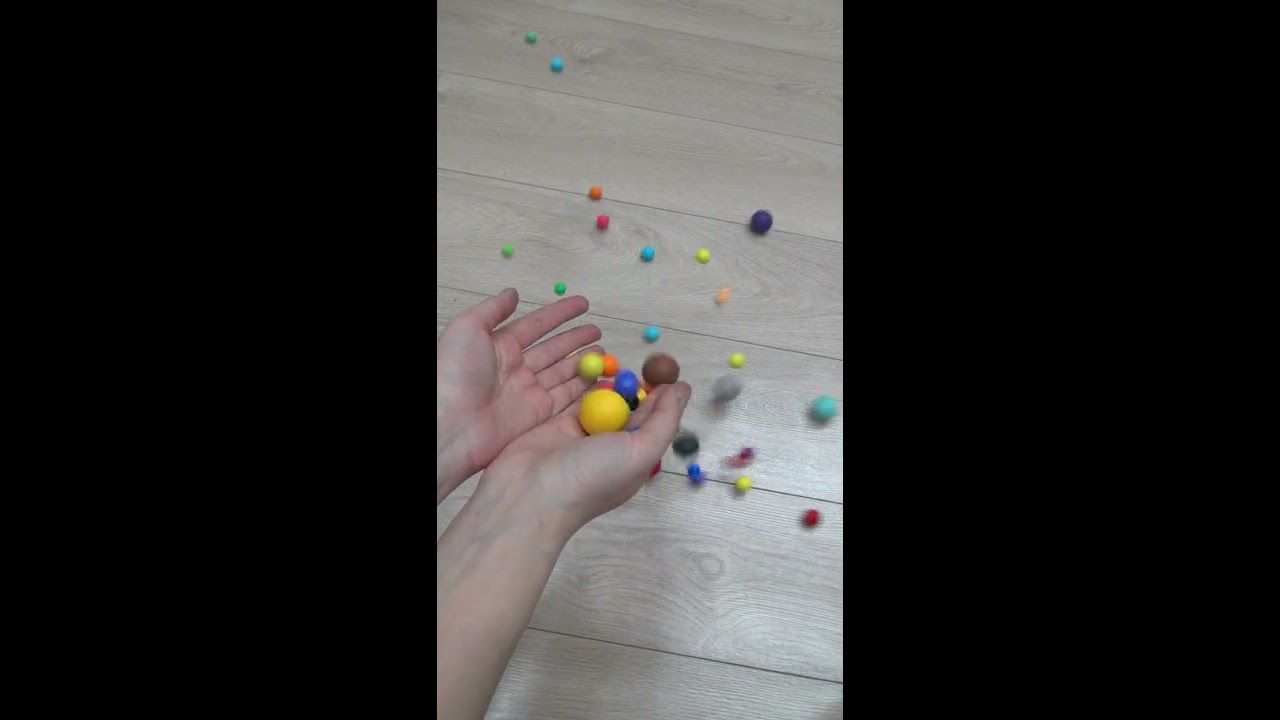The photograph is a horizontal rectangle with black borders on both sides, framing a narrow vertical section in the center where the activity is concentrated. The image is a close-up of two adult hands with light skin and visible blue veins, emerging from the bottom left corner. The palms are facing up, holding a collection of five to six small, colorful balls, with some larger than marbles but no bigger than ping pong balls. Each hand cradles different colors, including yellow, blue, orange, pink, and brown. On the wooden floor below, which has a light grayish-brown tint, numerous other balls are scattered. These balls are in various colors including red, blue, dark blue, gray, and orange, with most of them clustered in the center and a few blurred. A couple of additional balls, green and blue, are visible towards the upper part of the photograph. The hands seem poised as if either gathering or releasing the balls onto the floor, adding dynamic movement to the central tableau.